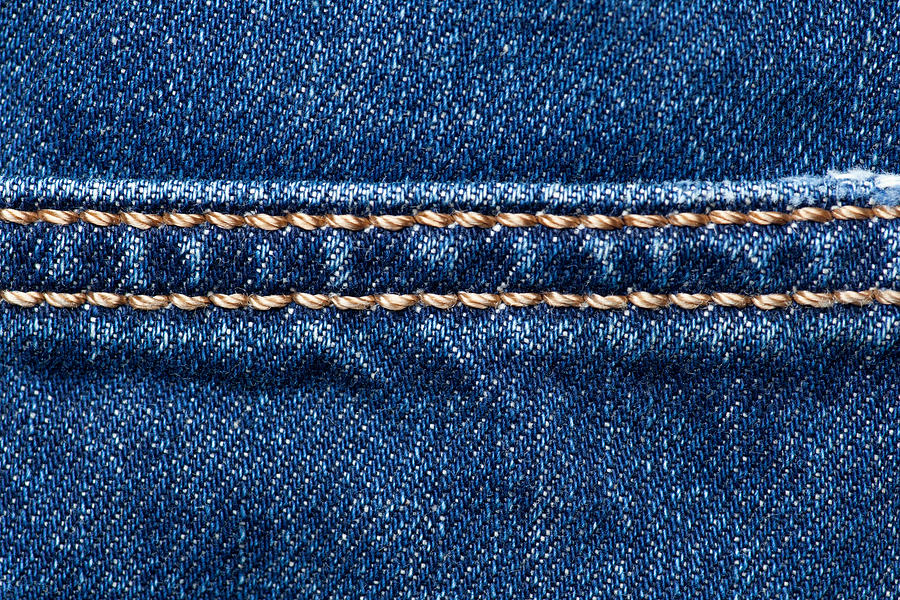This is a highly detailed, close-up image of a denim garment, most likely a pair of jeans. The denim fabric is a dark, rich blue with white speckles and variations in texture that give it a mottled appearance. The image focuses heavily on the stitching, showcasing two parallel rows of gold or light brown seams running horizontally. The stitching resembles golden braids and starts at the top left corner, extending continuously across the image to the right. The two seams are roughly an inch or less apart. Above these seams, there is a lighter, whitish stitching that may represent the edge of a pocket. The fabric below the first seam displays a slight puffiness, following the contour of the stitching. The entire image is rectangular and lies horizontally, capturing the intricate details of the denim texture and stitching.